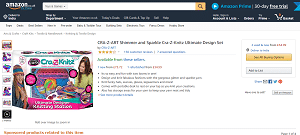The image appears to be a cluttered web interface, possibly from a mock-up or a glitching screenshot. Central to the image is an Amazon search bar featuring a black search icon enclosed within a yellow square. This is followed by numerous repetitive placeholder texts labeled "Blerr," both in the search bar and scattered throughout the rest of the interface.

Adjacent to the search bar is a location icon, equally accompanied by repeated instances of "Blerr." Further to the right, there is a shopping cart icon with an orange item inside, again annotated with "Blerr."

The middle section features a prominently labeled box "Crap Kids," depicting two children—one on the left and the other on the right of the box. The box is designed with two pink circles and a rainbow-colored beach ball on the front. Surrounding this feature are additional segments filled with the word "Blerr."

Below, there are four orange circles adjacent to further "Blerr" text in blue and green tones. Continuing downward, the visuals include two red elements also tagged with "Blerr," followed by a lengthy paragraph of the same placeholder text.

Towards the bottom right, there is an orange button labeled "Blerr" next to a gray button carrying the same inscription. The image finishes with more "Blerr" text at the bottom, along with an orange and black "Blerr" situated at the bottom right corner.

Overall, the image appears to be a mix of functional web elements overlaid with placeholder text, suggesting an unfinished or error-prone web design.